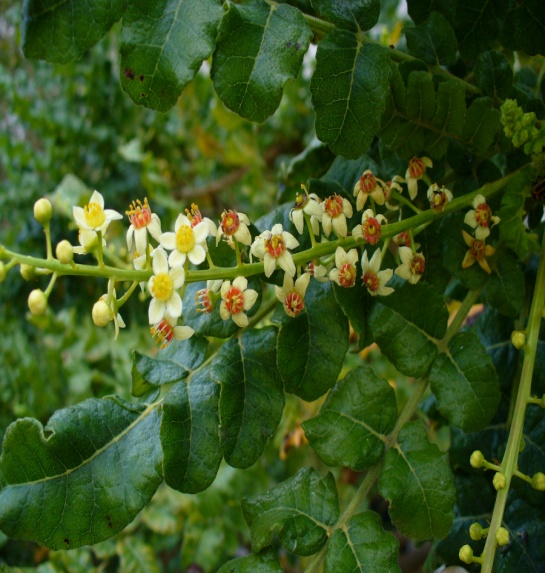The photograph showcases a detailed view of a plant, specifically focusing on the flower buds. The primary branch, adorned with vibrant green leaves, stretches across the image with a composition of three other prominent branches—one extending from the top right towards the left, and two descending downward. The leaves are predominantly healthy green, albeit with a few brown spots, highlighting the plant's overall vitality. The buds, some fully open and others partially bloomed, are intricately arranged along the central stem and various smaller branches. These flowers display delicate white petals surrounding either red or yellow centers, adding a vivid contrast to the lush greenery. The backdrop features more branches and flowers, amplifying the natural beauty of the scene. The atmosphere is subtly hazy, suggesting a morning setting, yet no human presence or textual elements distract from the plant’s organic splendor. The photographer has skillfully captured the essence of this serene and vibrant botanical moment.